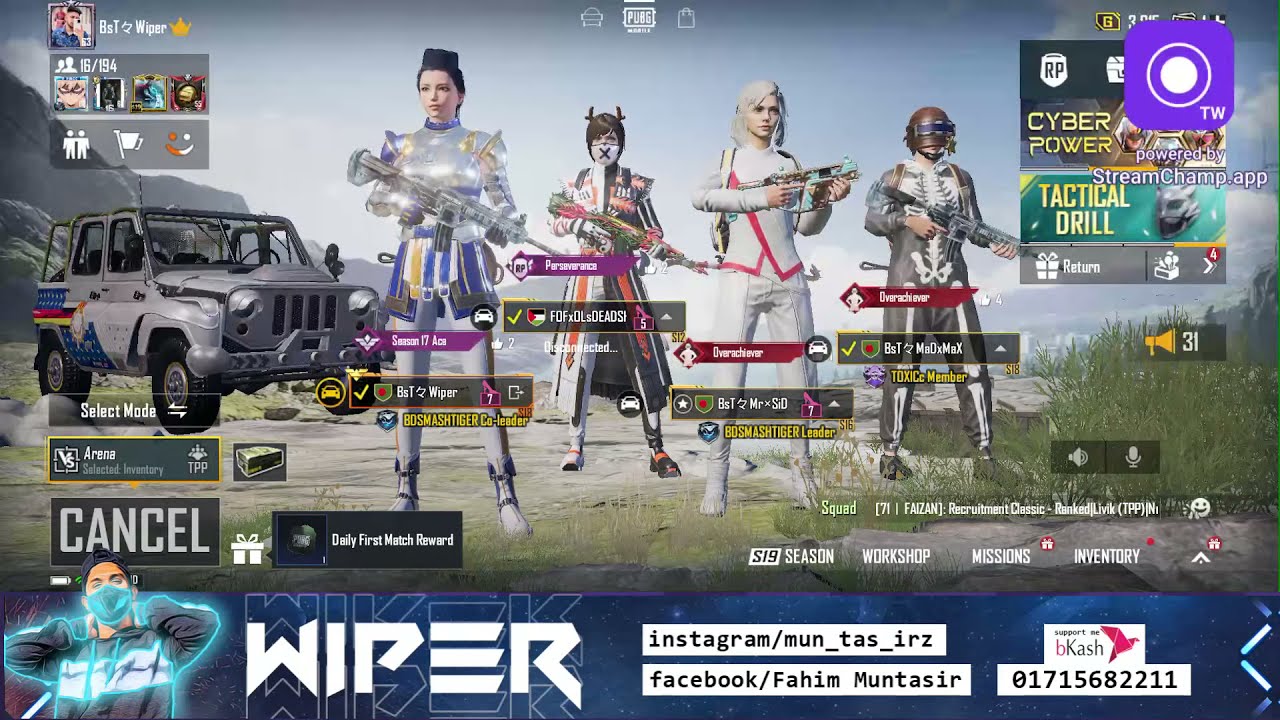The image appears to be a screenshot from a battle royale-style video game, showcasing a team of four characters, each wielding weapons and adorned in vibrant, distinctive outfits. The characters are standing on a sandy, rocky terrain, with a gray jeep positioned to the left side of the image. The first character wears intricate armor with a blue skirt and black hair. The second character sports an orange and white long jacket with small antlers on her head. The third character is dressed in white leather pants and a white leather jacket embellished with pink seams. The fourth character is clad in a black and white skeleton onesie, topped with a helmet featuring a blue-purple visor.

The bottom portion of the screen features a prominent banner that reads "WIPER" and displays Instagram (mon_taught_tasks_IRZ) and Facebook (Fahim Muntasir) addresses. Accompanying the social media links is a message encouraging support, along with a contact number (017-156-82-211). There are several other in-game interface elements, including "S-19 season," "workshop," "missions," and "inventory," contributing to a busy, text-heavy appearance. The bottom left corner also contains a gray cancel button.